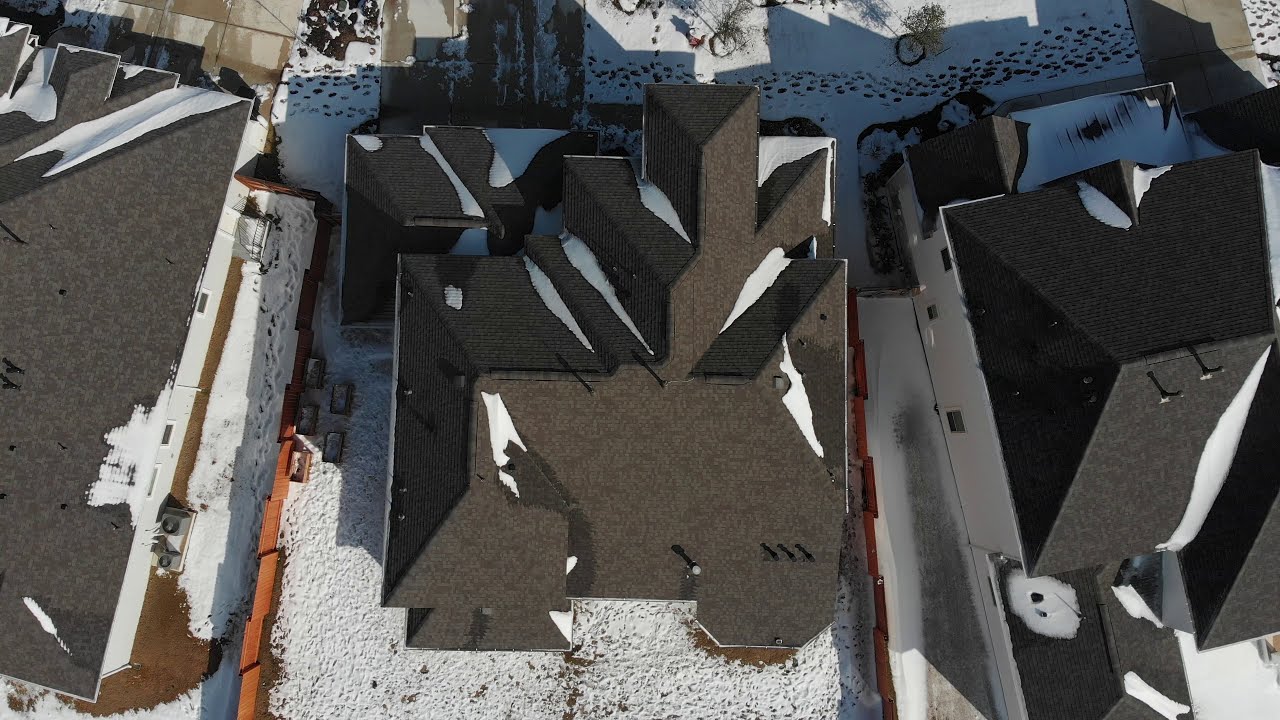This aerial photograph, taken in landscape mode on a clear day, centers on the roof of a house. The dark gray roof, segmented with snow in its cracks and crevices, exhibits a sharp angle and is punctuated by several steam pipes indicative of kitchen and bathroom vents. Surrounding the main house, which commands the center of the image, are neighboring houses with darker black roofs. To the right, the house features a white facade, while the house on the left has a white upper story and a red brick lower story. The snow-covered yard displays visible footprints leading from one sidewalk to another, nestled between the houses. Additionally, each house has air conditioning units along its sides. A partial shadow from an adjacent building creates a mix of lighter and darker patches on the roofs, enhancing the visual complexity of this detailed snow-laden scene.